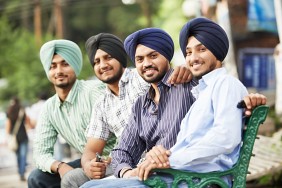In a vibrant and sunny park setting, four cheerful Sikh men are sitting in a row on a green, ornate metal bench, smiling warmly at the camera. Behind them, a backdrop of trees and a faint structure adds to the idyllic outdoor environment. Each man wears a distinct turban, ranging in color from mint green to black and two in dark navy blue. Their attire consists of casual work shirts: the man on the far left sports a long mint green shirt, the one next to him is clad in a short-sleeved checked shirt, the third wears a long-sleeved navy blue shirt with stripes, and the fourth man dons a light blue shirt. Amid the relaxed atmosphere, one of the men is holding something black and cylindrical in his hands, contributing an air of curiosity. The camaraderie among them is palpable, making it a delightful and engaging photo filled with positive, happy vibes.